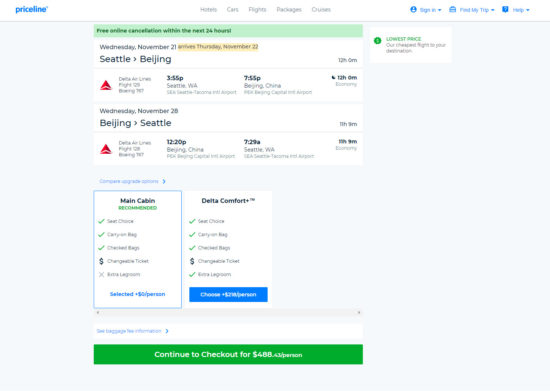The image captures a detailed view of a travel booking webpage. At the very top, there's a white header. On the left side of this header, the word "priceline" is displayed in small, light blue, lowercase letters. To the right of this, a navigation menu lists options for "Hotels," "Cars," "Flights," "Packages," and "Cruises." Further to the right, there are three prominently colored buttons: a blue "Sign In" button, a blue "Find My Trip" button, and a blue "Help" button.

Below the header, there's a green box featuring the message "Free online cancellation within the next 24 hours" (though the text is somewhat blurry). The webpage then lists travel details starting with "Wednesday, November 21st," indicating an arrival on "Thursday, November 22nd." The planned route is from Seattle to Beijing. The airline logos and the text "Delta Airlines" are visible alongside an unreadable flight number. It mentions a departure at "3:55 PM" from Seattle, Washington, arriving at "7:55 PM" in Beijing, China.

Following this, the return details are noted as "Wednesday, November 28th" (text slightly unclear), detailing the trip from Beijing back to Seattle. The return flight departs at "12:20 PM" from Beijing, China, and arrives at "7:29 AM" in Seattle, Washington.